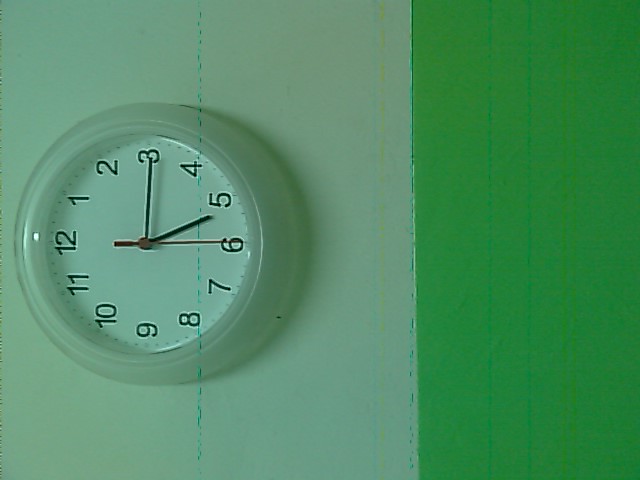This photograph depicts a round wall clock with a white face encased in a light greenish-gray plastic or glass material. The clock is oriented horizontally, with the numbers 12 and 6 positioned along a horizontal line from left to right. The clock shows the time as quarter past five, with the black hour and minute hands pointing to 3 and 1 respectively, and the black second hand at the 30-second mark or the 6 position. Despite the predominantly green hue cast over the image, likely from a green lens or shadow, the clock's clear plastic casing is partially reflective under the dim lighting. The clock is mounted on a wall that is divided into two distinct color sections: a light grayish-green that occupies two-thirds of the left side and a vibrant grass green on the remaining right side. Additionally, there is a small, noticeable imperfection in the form of a dotted line intersecting the clock face at the 8 and 4 positions, extending from the top to the bottom of the photograph.